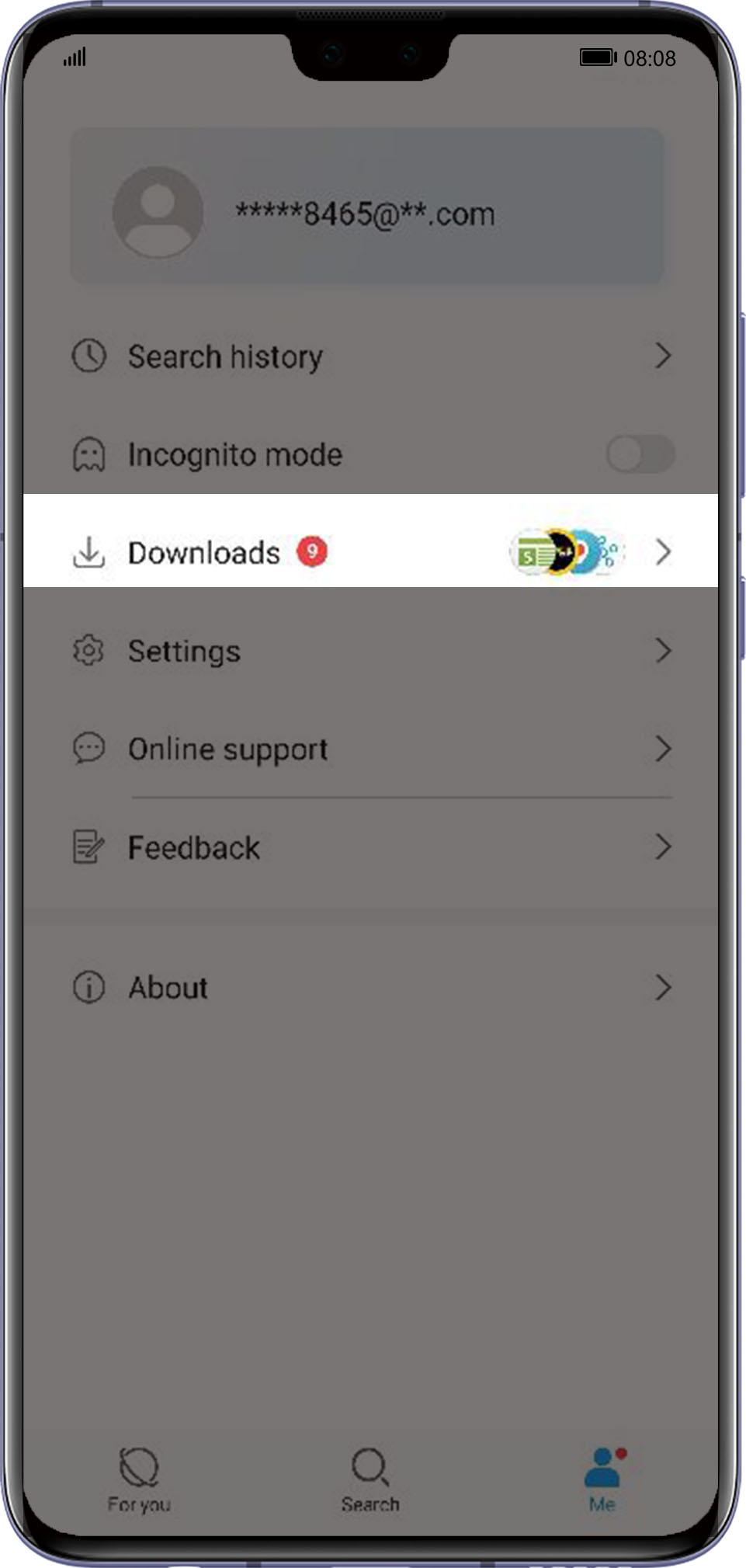A detailed photograph of a mobile phone showing its entire physical frame against a neutral background. The screen displays an active call with a phone number partially dialed and visible at the top. Below this, there is a section labeled "Downloads" which is highlighted and contains nine distinct download options. The time displayed on the phone is 8:08 PM, and the battery icon indicates a full charge. The rest of the screen appears slightly grayed out, drawing focus to the highlighted areas.